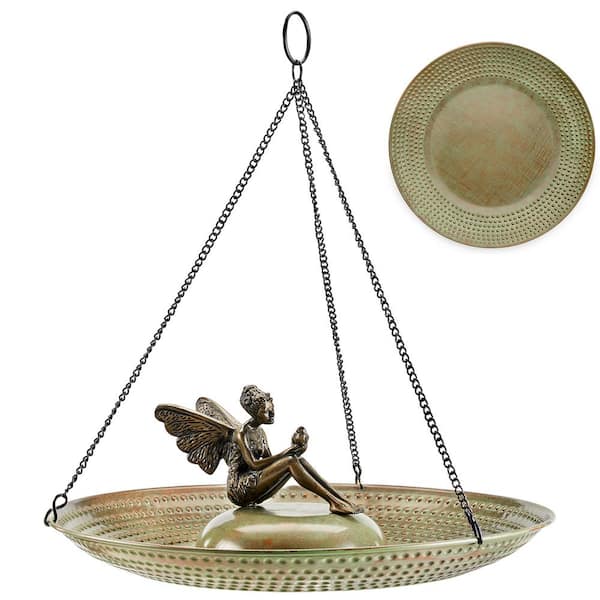The image features a detailed close-up of a hanging, gold-colored decorative dish, resembling an ornate fruit holder or scale. The dish's shallow depth is adorned along the rim with circular, textured designs and layers of bumps, giving it a vintage, almost timeworn appearance with spatterings of green and copper hues.

Central to this piece is a small, raised dome, also exhibiting a green and copper patina, on which a intricately sculpted fairy or angel figure is perched. The fairy, adorned in a delicate dress, sits with her legs stretched out but bent at the knee, and is positioned facing the right side of the image. She has wings on her back and is holding a small, round object, possibly an acorn or a tiny jar, gazing at it with a caring expression.

This detailed sculpture is suspended via three chains that connect from the dish to a central ring, allowing the entire piece to be hung up. On the right-hand side of the image, an alternate view of the dish, seen from the top down, accentuates the textured decorations and highlights the item's intricate craftsmanship and aged charm.